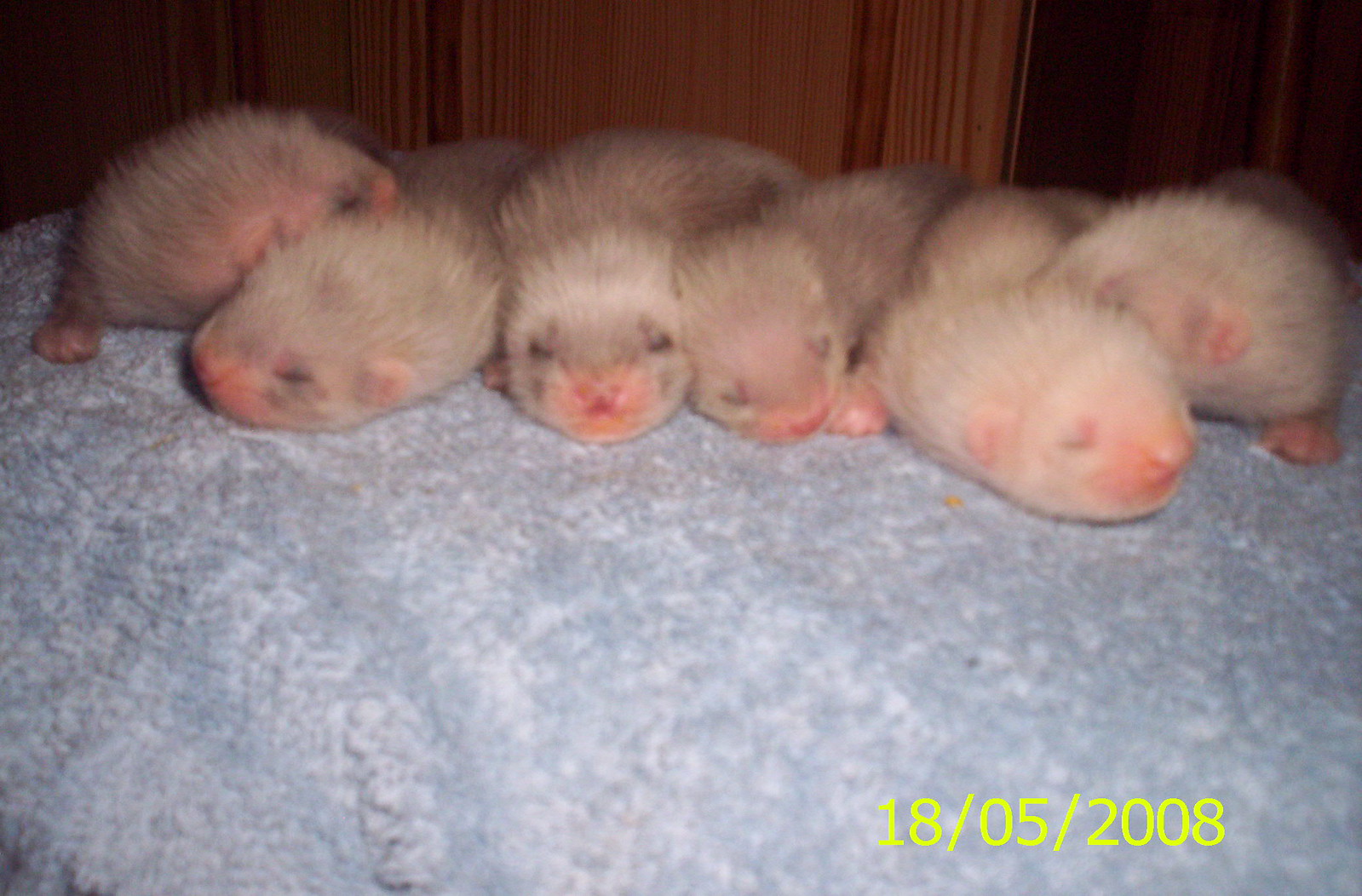The image features six adorable baby ferrets with creamy white fur and dark eyes, peacefully asleep on a light blue and white cover, which has a fluffy and soft texture. Their tiny pink ears stick up from the sides of their heads, and their pink noses and mouths add a touch of cuteness to their faces. The ferrets, lined up in a row with their eyes closed, showcase their short legs and small paws. Behind them, wooden panels suggest a rustic background, possibly part of a Chesterfield case. In the bottom right corner, the date "18/05/2008" is displayed in bright lime green font, signifying the time the photograph, which seems to be of low quality possibly taken with an early digital camera, was taken. The overall scene captures the endearing innocence of the baby ferrets, creating a charming and heartwarming image.